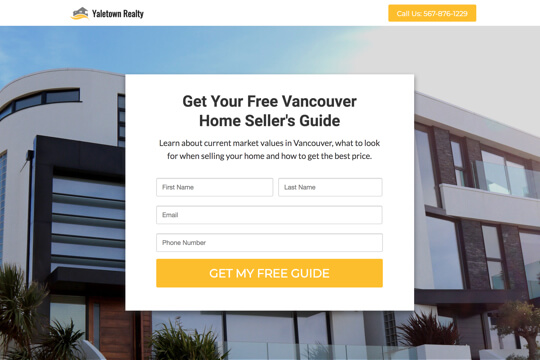This image is a detailed screenshot of a website's homepage. Dominating the top of the page is a white header. Situated on the left side of this header is a gray house icon with a yellow wave beneath it. To the right of the icon, the website's name, "Yale Town Realty" is displayed in black text, with both the 'Y' and 'R' capitalized.

In the top right corner of the header, there's a yellow rectangular button with slightly rounded corners. This button features white text that reads, "Call Us 567-876-1229."

The main body of the webpage features a background image of a contemporary building. The building has a predominantly white façade with accents of dark gray stone, black sections, and reddish wooden elements. In front of the building are small green bushes, and the sky above is a gradient of blue that fades into white towards the top right corner.

Superimposed onto this background is a white pop-up window. Centered at the top of the pop-up is a bold black text that reads, "Get Your Free Vancouver Home Seller's Guide." Below this, two lines of smaller black text provide additional details: "Learn About Current Market Values in Vancouver, What to Look For When Selling Your Home, and How to Get the Best Price."

The pop-up contains three rows of text input boxes. The first row features two nearly equal-sized boxes labeled "First Name" and "Last Name." The second row has a single text box labeled "Email," and the third row has another single text box labeled "Phone Number." All text boxes have a thin light gray outline and placeholder text in light gray.

At the bottom of the pop-up is a wide yellow button with sharp corners. The button's white text is in all caps and reads, "Get My Free Guide."